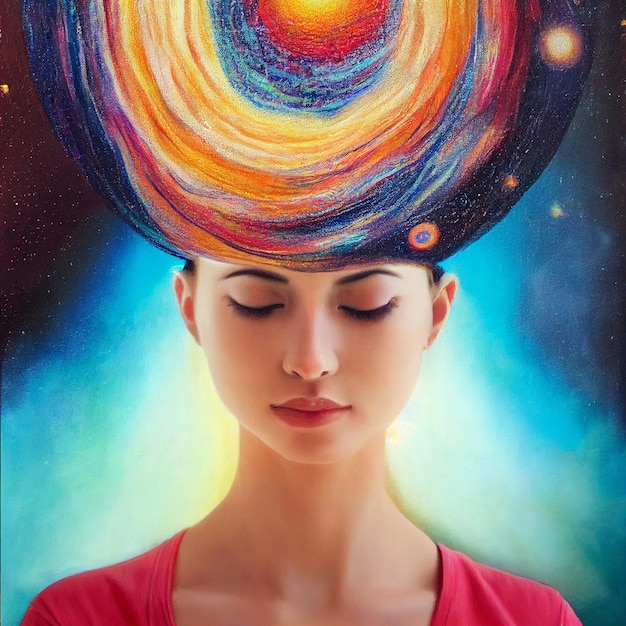The digitally altered image depicts a woman with closed eyes, facing downward. She has darkened eyebrows, red lipstick, and wears a pink shirt. Her head is adorned with a vibrant, galaxy-like spiral of colors, including yellow, red, blue, and orange, replacing her hair. The background features a space-themed scene: on the left, a deep black sky filled with small stars; on the right, a blue-tinted expanse with tiny specks representing stars and a gaseous glow beneath. The area around her skin transitions from a gradient of dark blue to white, with a warm yellow halo effect near her face and neck, enveloped in an array of starry and colorful nebulous clouds. The image's atmosphere is surreal, as if blending cosmic wonder with human presence.